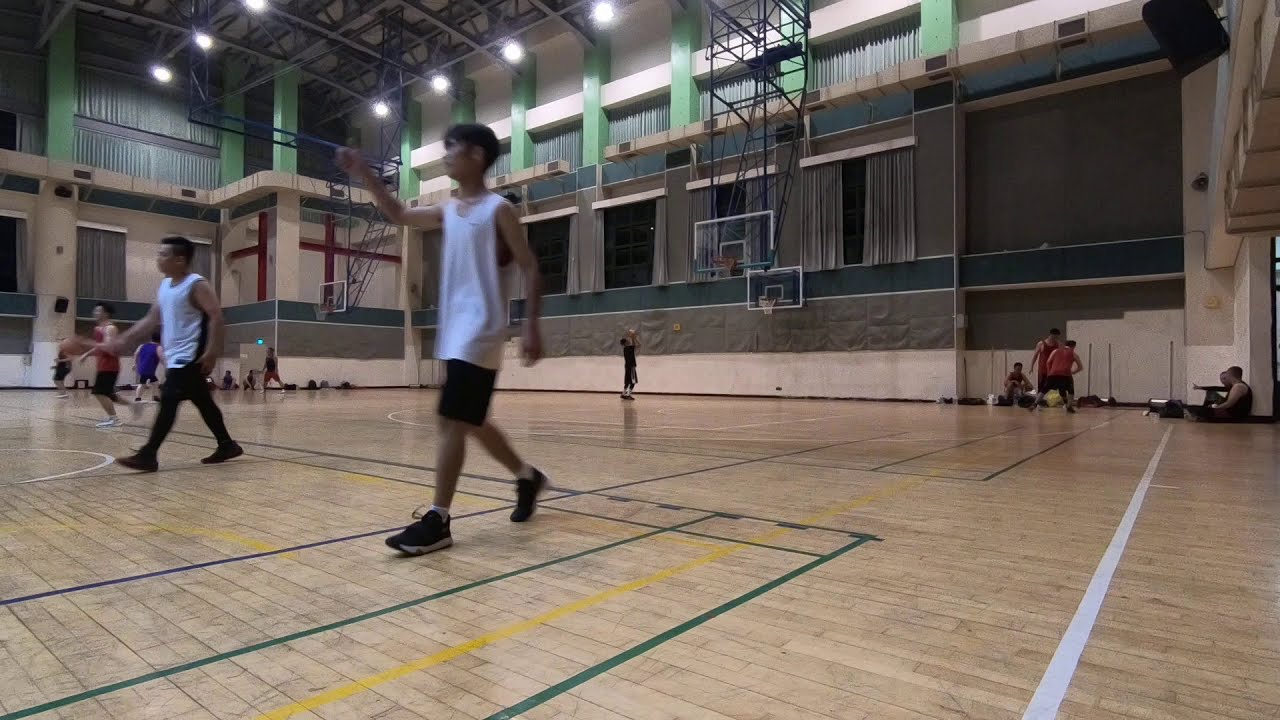In this indoor gymnasium, we see several men engaged in a lively basketball game on a hardwood court. The gym features towering ceilings, likely over 50 feet high, adorned with bright white lights. Green pillars and white horizontal structures line the walls, adding to the gym's spacious feel. The court itself is marked with taped sections in green, yellow, and blue, and lit by overhead lights.

At the center of the scene, a man dressed in all black is captured mid-shot, aiming for one of the two hoops that descend from the ceiling. Another player is seen in a maroon tank top, dribbling the ball, facing left. A few players sporting white tank tops can also be seen; one wears black shorts and shoes while another is in black pants and shoes.

On the sidelines, a mix of seated and standing spectators line a white wall, their attention fixed on the game. The far side of the court hosts additional onlookers, all under the watchful gaze of the overhead lights. The colors scattered throughout the scene include tan, green, yellow, red, purple, white, black, brown, and silver, creating a vibrant atmosphere in this well-lit and dynamic setting.